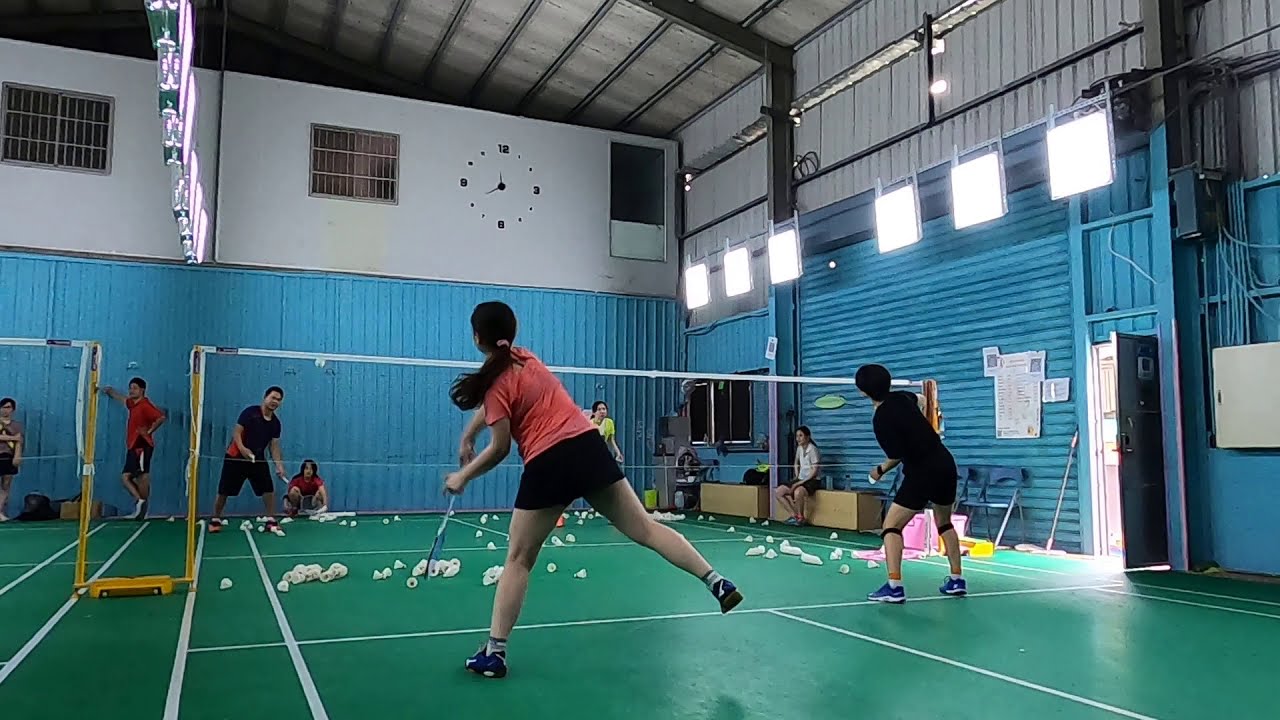This is an indoor scene depicting a recreational badminton game in progress, possibly a two-on-two match involving several girls. The green court is marked with yellow lines and spans the image with a white net supported by yellow structures crossing the middle. The walls of the stadium are light blue, resembling blue paneling or shutters, and feature a prominent clock that reads approximately 11:35. The ceiling is white, with hanging lights positioned on the top left, top right, and center. 

In the foreground, two girls are playing. One, wearing a red t-shirt and black shorts with long hair tied up, has just served. The other player, dressed in a black t-shirt and black shorts, with short hair and knee supports, appears ready to return the serve. Across the net, two more participants, also in black t-shirts, are preparing for the shot, while a man and another girl are positioned as observers or participants. Additionally, there's a girl sitting on the ground and another preparing to receive a serve.

The background includes a wall clock and an open door on the right, letting in natural light. Several shuttlecocks are scattered on the court, hinting at ongoing practice or multiple serves. The scene is lit by both the artificial lights and natural light entering from the door. Various electrical wires and boxes can be seen alongside the walls, adding to the detailed indoor setting of the recreational sports area.